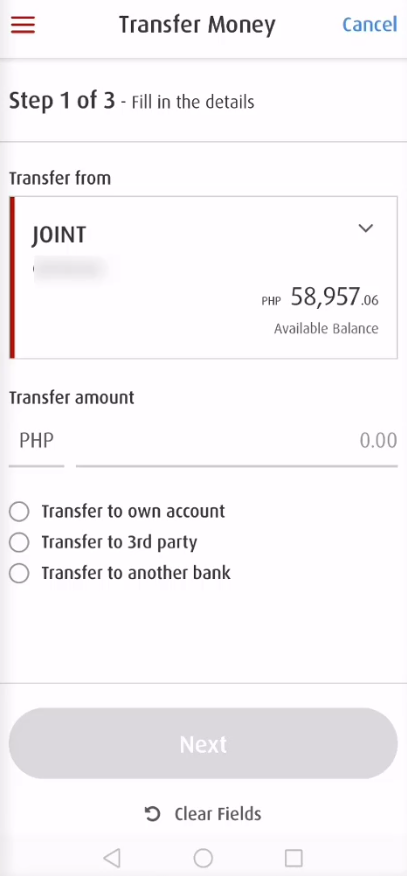The image displays a mobile banking interface with a white background. In the top left corner, there are three horizontal red lines, indicating a menu icon. At the center-top, the text "Transfer Money" is written in black, and directly to the right, a blue "Cancel" button is visible. 

Below this, the text "Step 1 of 3: Fill in the details" is displayed. Under this header, the section for "Transfer From" is marked in black text with a red vertical line to its left, indicating the selected account. The account type is labeled "Joint", accompanied by a downward arrow for additional options, and shows an available balance of PHP 58,957.06. 

Next, a "Transfer Amount" field is set to PHP 0.00 by default. Below this, there are options for transferring funds: "Transfer to Own Account," "Transfer to Third Party," and "Transfer to Another Bank." There's a "Next" button to proceed to the following screen and an option to "Clear Fields" accompanied by a back arrow.

At the bottom of the interface, typical navigation icons for a back triangle, circle, and square are present. The overall design is clean and straightforward, ensuring users can navigate and complete the transfer process with ease.